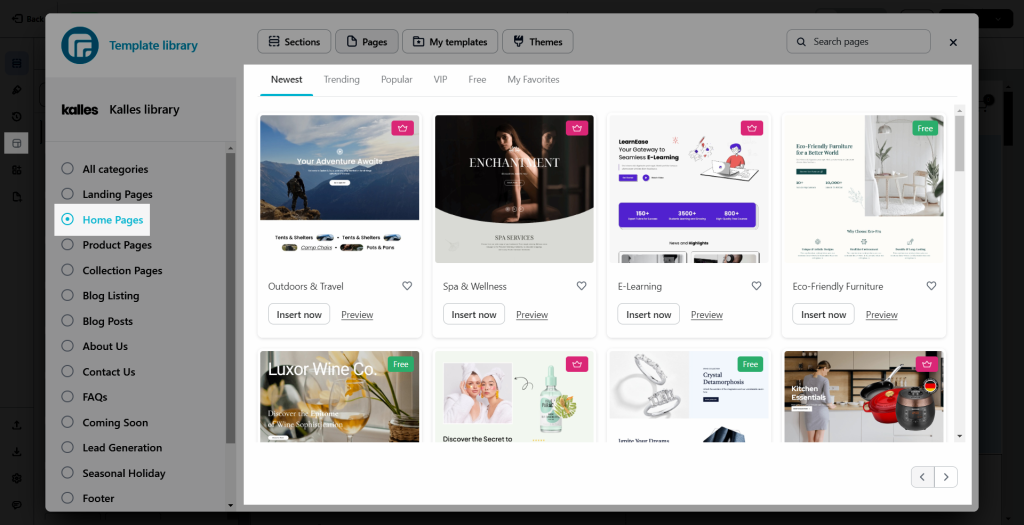This screen capture appears to be taken from a monitor, not a cell phone, with a background that blends gray, white, and black hues. There's an active pop-up window causing the background text to appear faded. In the upper left-hand corner of this muted gray area is a blue icon accompanied by the text "Template Library" in blue. Directly beneath it, in bold lettering, is "KALLES KALLES Library."

An open menu is displayed on the left side, featuring radio buttons next to labels such as "All Categories," "Landing Pages," "Home Pages," "Product Pages," "Collection Pages," "Blog Listing," "Blog Post," "About Us," "Contact Us," "FAQs," "Coming Soon," "Lead Generation," and "Seasonal Holiday and Footer." The "Home Page" option is selected, making it appear vivid blue against a white background.

On the right-hand side, the open window showcases various design offerings. At the top, tabs labeled "Newest," "Trending," "Popular," "VIP," "Free," and "My Favorites" are visible. Below these tabs are two rows of web page designs arranged horizontally. These designs range from outdoorsy themes to luxury looks and minimalist styles, including specific sites like a wine site and a jewelry site. None of the designs have been selected yet. Designs marked as free are highlighted in green with white lettering indicating "Free," while others feature a pink icon with a white flower outline, suggesting these templates require purchase.